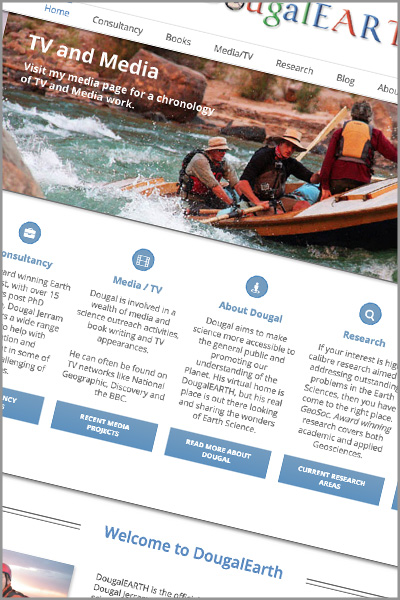This image is a cropped screenshot of a tilted website, giving the entire scene an angled appearance, despite the image itself being square. Surrounding the image is a dark gray border of around two to three pixels in width. Starting from the top right corner and moving diagonally, the partial letters "U-G-A-L" in lowercase and "E-A-R" in uppercase are visible, suggesting the word "Earth" with alternating blue and red letters.

Beneath this is a thin dividing line, also slanted at an angle of approximately 20 to 30 degrees. Below this line is a navigation menu, aligned diagonally, listing the following links in order: Home, Consultancy, Books, Media, TV, Research, Blog, and the word "About" cut off due to the image's edge.

In the banner section directly below, an image of three men white water rafting through what appears to be a canyon, possibly the Grand Canyon, is featured. Superimposed in large, white sans-serif text is "TV and Media". Below this heading, in smaller text, the caption reads: "Visit my media page for a chronology of TV and media work."

Further down, on a white background, there are four information boxes. Each box contains an icon at the top, a subheading, a paragraph of text, and a button at the bottom, all slightly tilted:

1. The first box partially visible, with a white suitcase icon inside a blue circle, appears to be labeled "Consultancy". The text and button are partially cut off due to the angle.
2. The second box, fully visible, features a film icon within a blue circle and the subheading "Media/TV". The text reads: "Dougal is involved in a wealth of media and science outreach activities, book writing, and TV appearances. He can often be found on TV networks like National Geographic, Discovery, and the BBC." This box also includes a button labeled "Recent media projects".
3. The third box, visible with partial text and a sliver of the subsequent button, is labeled "About Dougal".
4. The fourth box is titled "Research", containing an icon at the top, descriptive text below, and a button at the bottom.

Beneath these boxes, a dividing line runs at the same angle. Centered between two horizontal lines, in blue letters, is the text "Welcome to Dougal Earth". At the very bottom of the image, a new picture begins alongside partial text, both nearly cut off by the cropped edge.

Overall, the distinctive angled presentation of this website capture imparts a dynamic, albeit somewhat skewed, visual narrative.